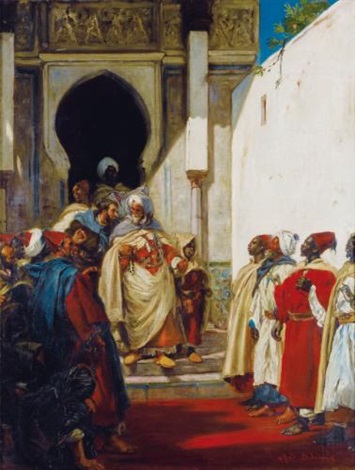The image depicts a detailed, artistic painting set in a historical Middle Eastern or African scene. Central to the composition is a grand, white building with a dark brown, intricately designed top, and an archway leading up through a set of steps. On either side of the archway, two white beams hang vertically down into pipes at the bottom. In the upper right corner, a sliver of blue sky framed by green foliage is visible.

In this scene, a group of people is gathered in front of the building, focusing around a prominent red carpet that divides them. Four individuals stand with their backs against the white wall. These include a person in a golden robe, another in a white robe, a third in a red robe with a white hat, and a fourth man standing in the doorway in a white turban. Adjacent to the doorway, an old man with a white turban and a robe interacts with a man leaning forward, whispering into his ear, who has brown hair and a short beard.

At the bottom of the steps, more individuals, some in white turbans and others in fez-style caps, stand at attention along the red carpet, highlighting the presence of a significant central figure. This main character, clad in a highly decorated red garment with a long white cloak, stands on the steps, engaging in conversation. The variance in skin tones among the people – from light-skinned to black Africans – adds diversity to the attire of robes and headgear, emphasizing the cultural richness of the setting.